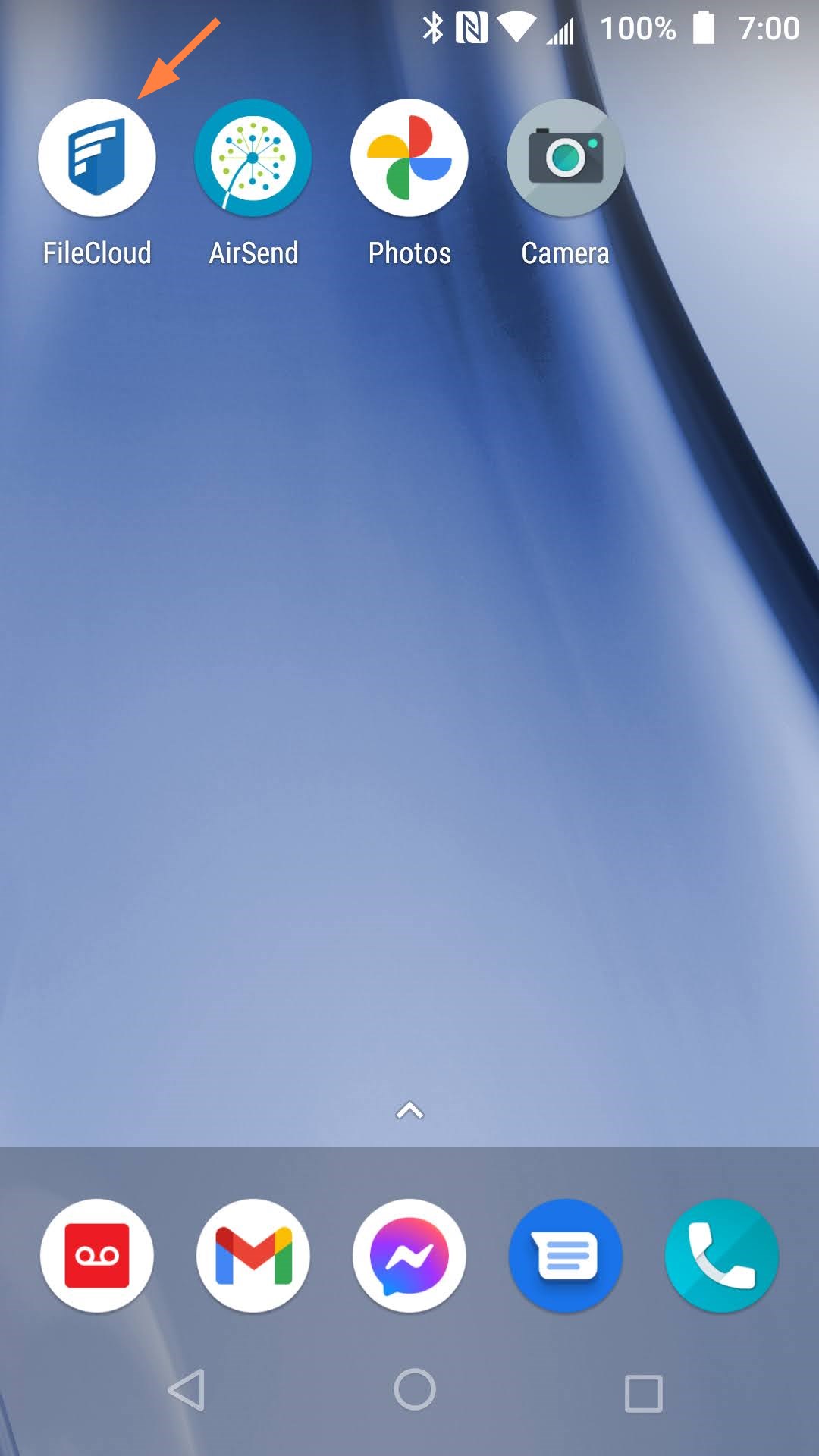The screenshot displays the top section of a smartphone's home screen. In the status bar, the Bluetooth and Wi-Fi icons are visible, alongside the signal strength indicator showing four bars, and a fully charged battery icon. The time is displayed as 7:00. 

A bright orange arrow points to an icon in the top-left corner, which consists of a white oval with a blue shield containing three white lines of varying lengths, labeled "File Cloud." Next to this is an icon of a blue clock labeled "AirSend."

Following this, there's an icon consisting of a white oval with interlocked red, blue, green, and yellow semi-circles, labeled "Photo." The next icon is a gray oval featuring a camera, labeled "Camera."

The background of the screen is a light blue, almost grayish, swirling pattern.